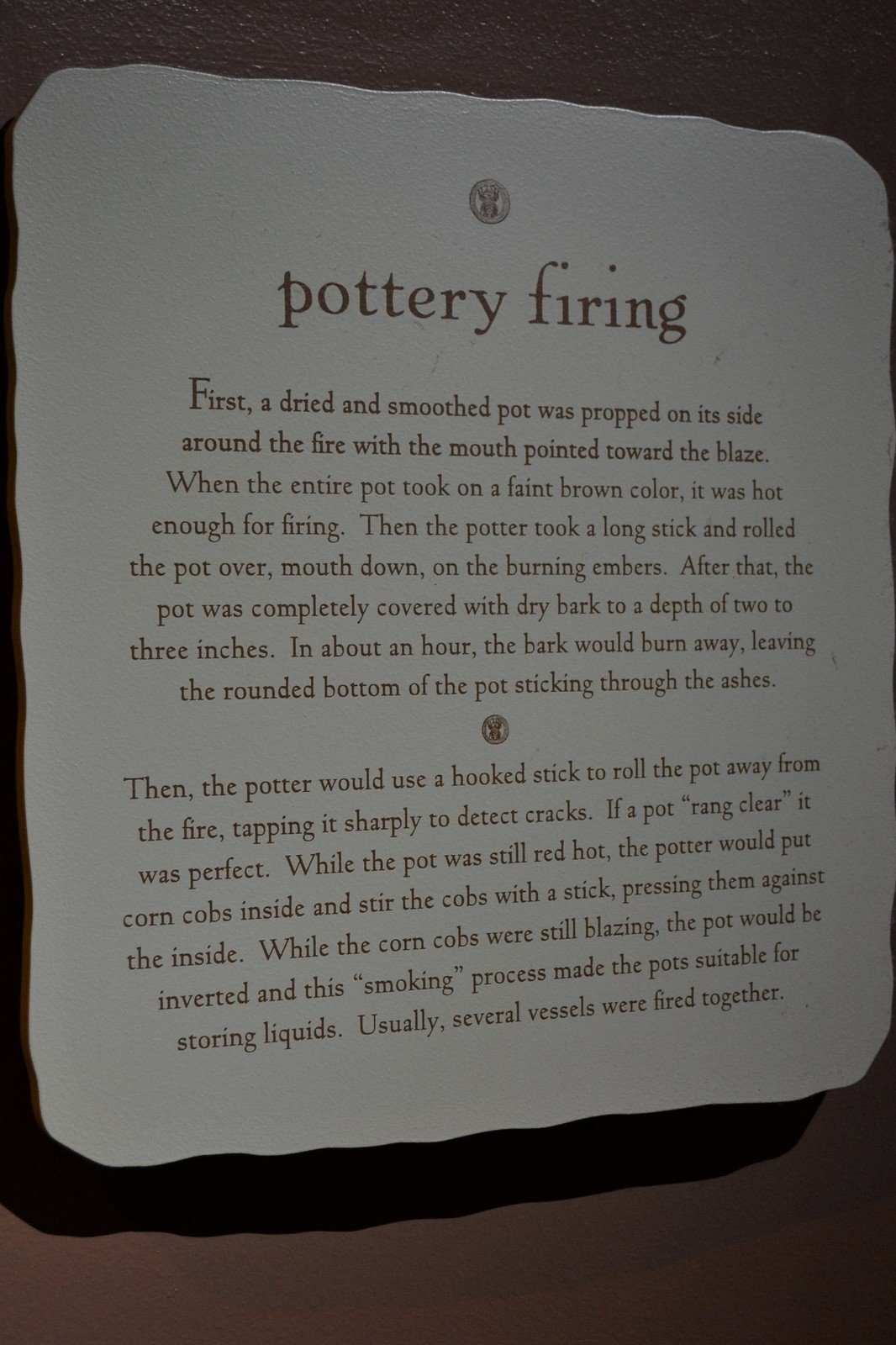The photograph depicts a white wall-mounted plaque with wavy, rigid edges and detailed bronze-colored lettering describing the process of pottery firing. Prominently titled "Pottery Firing" in larger letters, the plaque outlines the traditional method in smaller text. It begins with, "First, a dried and smooth pot was propped on its side around the fire with the mouth pointed toward the blaze. When the entire pot took on a faint brown color, it was hot enough for firing. Then the potter took a long stick and rolled the pot over, mouth down on the burning embers. After that, the pot was completely covered with dry bark to a depth of two to three inches. In about an hour, the bark would burn away, leaving the rounded bottom of the pot sticking to the ashes." 

Below this initial paragraph is a circular emblem or logo, followed by another section of text that describes the subsequent steps: "Then the potter would use a hooked stick to roll the pot away from the fire, tapping it sharply to detect cracks. If a pot rang clear, it was perfect. While the pot was still red hot, the potter would put corn cobs inside and stir them with a stick, pressing against the inside. While the corn cobs were still blazing, the pot would be inverted, and this smoking process made the pot suitable for storing liquids. Usually, several vessels were fired together."

The background of the plaque contrasts sharply as it is mounted against a dark brown or almost black wall, which enhances the visibility of the text and its artistic presentation.